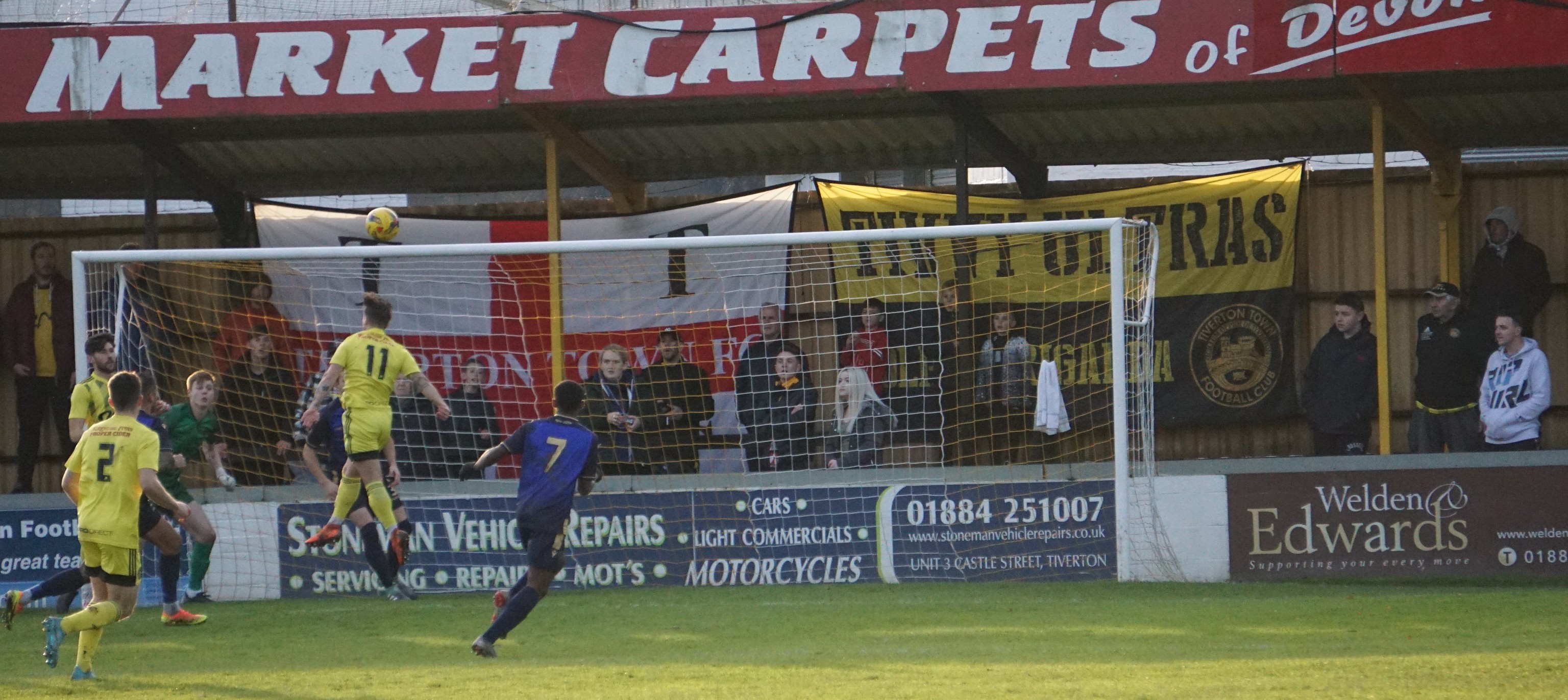In this vibrant, action-filled photograph of a soccer match, we see a grassy field in the foreground, with the scene centered around a goal post. The intense, midday outdoor setting highlights several players in motion. Three players clad in yellow jerseys, shorts, and socks, one player in a blue jersey with black shorts, and another in green complete with matching apparel, all vie for the ball. The action focuses on one of the yellow-clad players, who is airborne, having just executed a header with the ball now suspended above him. The white net and white posts of the goal frame the scene where the players' backs face the photographer.

In the background, we observe a wall lined with advertisements and a crowd of spectators keenly watching the action. Above the spectators, banners are prominently displayed, including a red banner with "mark it carpets" written in white letters, alongside other promotional signage. The vivid colors in the image – the green of the field and the player's jersey, the yellow uniforms, blue and black clothing, and the multicolored advertisements and banners – all contribute to the dynamic atmosphere of this soccer match in play.